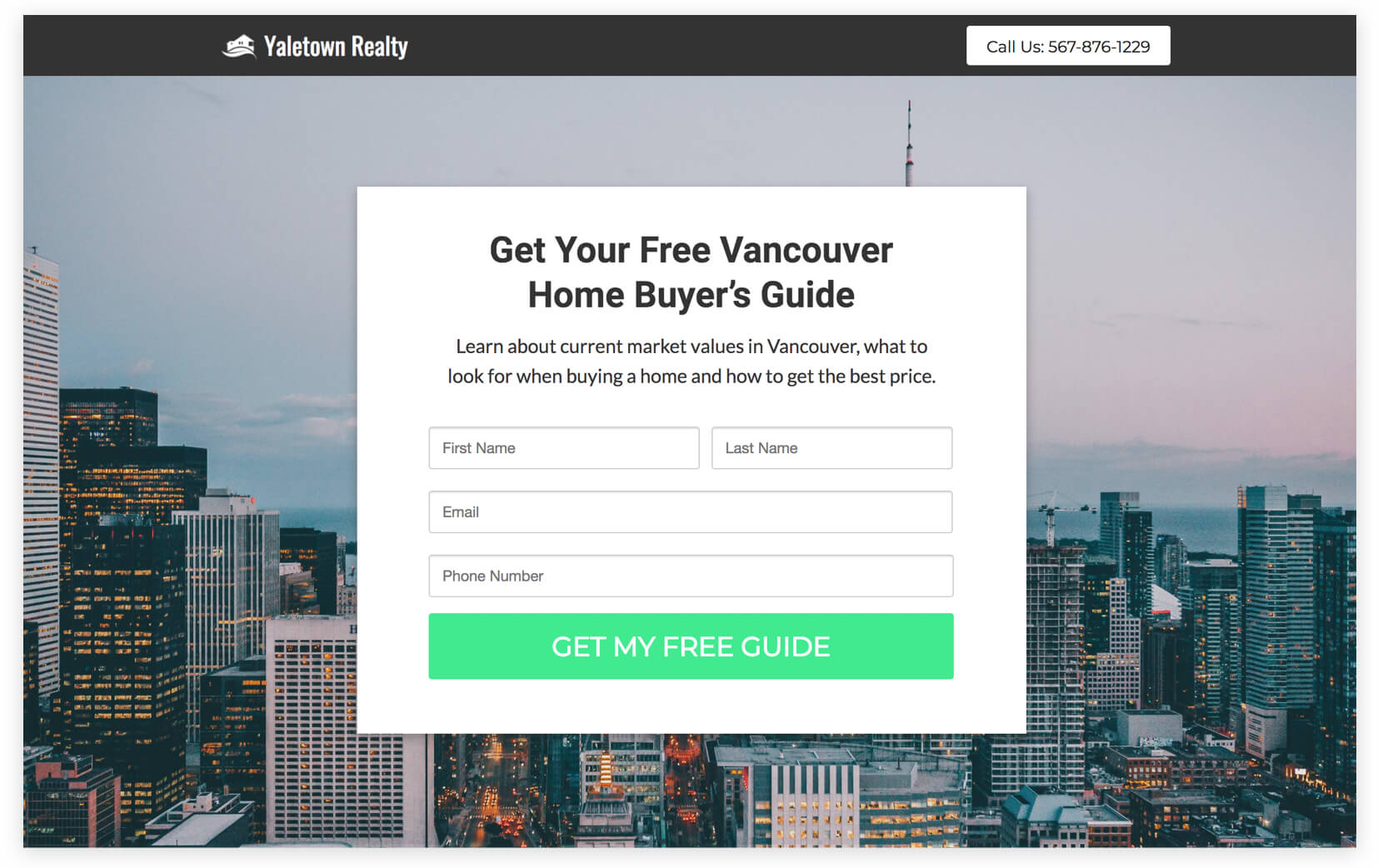The image depicts the Yaletown Realty website. At the top of the page, "Yaletown Realty" is prominently displayed, adjacent to a black banner positioned on the left side. To the left of the banner, there's an icon resembling a house. On the right-hand side of the page, a rectangular box contains the text "Call us: 567-876-1229".

The background features a cityscape, potentially a downtown area of Vancouver, captured during the evening. The cityscape showcases large buildings with illuminated windows, giving the scene a vibrant feel.

Centrally placed on the webpage is an overlay with bold black font, announcing: "Get your free Vancouver home buyers guide," centered on the page. Below this, the text provides additional details: "Learn about current market values in Vancouver, what to look for when buying a home, and how to get the best price."

Beneath this section, there is an input box for the first name on the left side, followed by another input box on the right for the last name, both aligned to the left. Below these, a long rectangular box is meant for email entry. Further down, there's a space followed by another rectangular box for the phone number. At the bottom of this form, a thick rectangular box, highlighted in green, urges users to "Get My Free Guide".